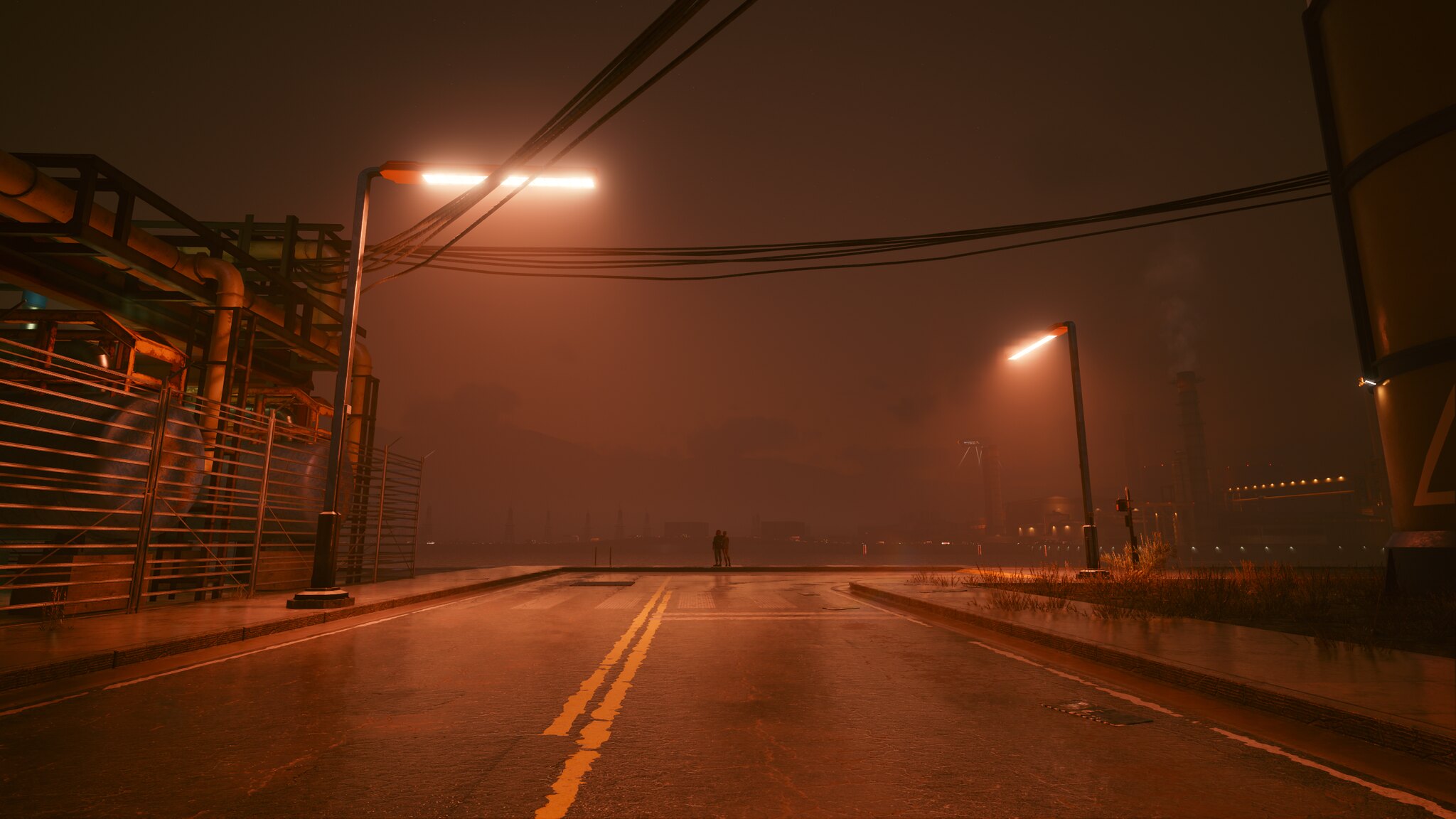A photograph captures an atmospheric scene drenched in thick fog or mist, likely taken outdoors with a standard camera. The image's center features a damp, wet roadway, reflecting the moisture in the air. The sky is obscured by heavy fog, adding a sense of mystique to the scene. A reddish overtone envelops the entire picture, possibly due to the lighting conditions at the time. Streetlights extend over the roadway, casting a glow that appears reddish despite their bright yellow-white emission.

Stretching across the scene, electrical or telephone lines can be seen running parallel along the bottom and then intersecting perpendicularly at the top. A lone man stands at the end of the road, his figure sharply contrasting against the foggy background. In the distance, a factory emits wisps of smoke, illuminated by numerous industrial lights. On the left side of the image, various mechanical structures and equipment are visible behind a fence, further contributing to the industrial ambiance.